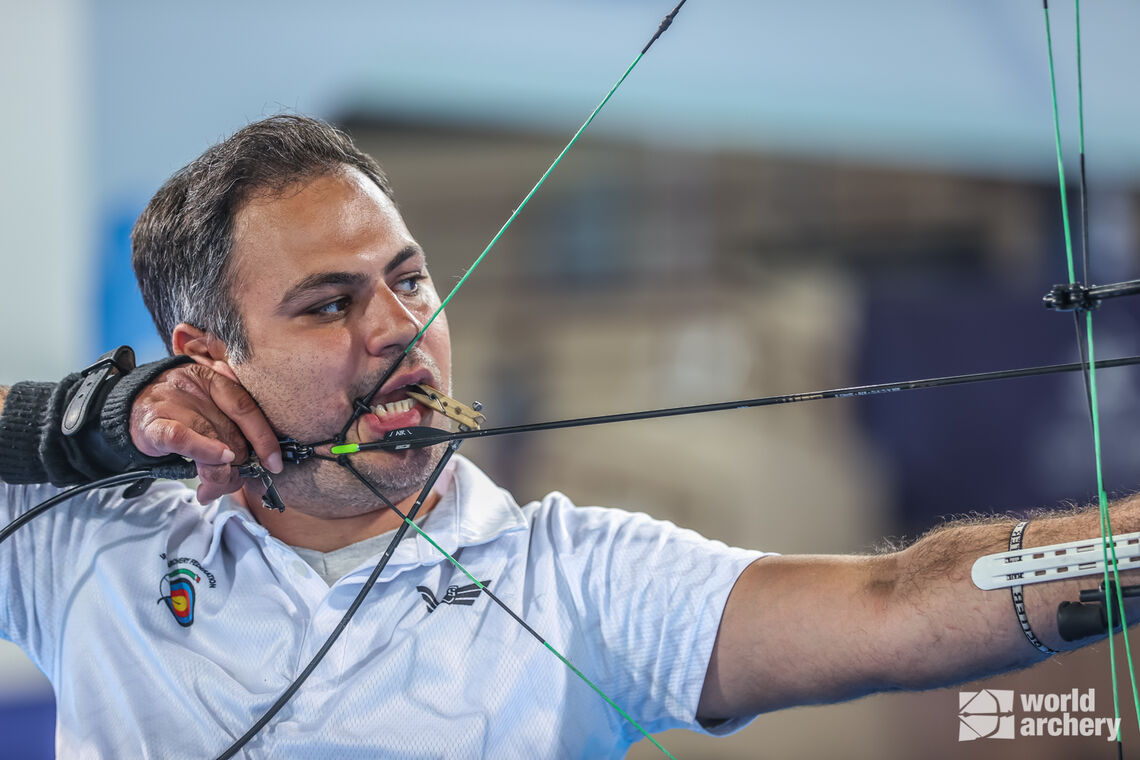This photograph captures an intense moment of an older male archer participating in a World Archery competition. The archer, with focused eyes locked on his target, is depicted to the left side of the frame, pulling the bowstring back to his cheek, with an arrow nocked but not fully visible. His right arm, clad in a black fingerless glove and adorned with a watch, is drawn back near his ear. His left arm is fully extended, holding the bow, and his slightly open mouth grips a clothesline attached to a cable. He wears a collared white shirt with a light blue hue that bears the World Archery logo and another, less discernible symbol in black. The background is artistically blurred, bringing the sharply focused contestant and his equipment to the forefront. In the bottom right, the World Archery logo and the words "WORLD ARCHERY" in white font enhance the professional quality of the image, emphasizing his dedication and the competitive nature of the sport.